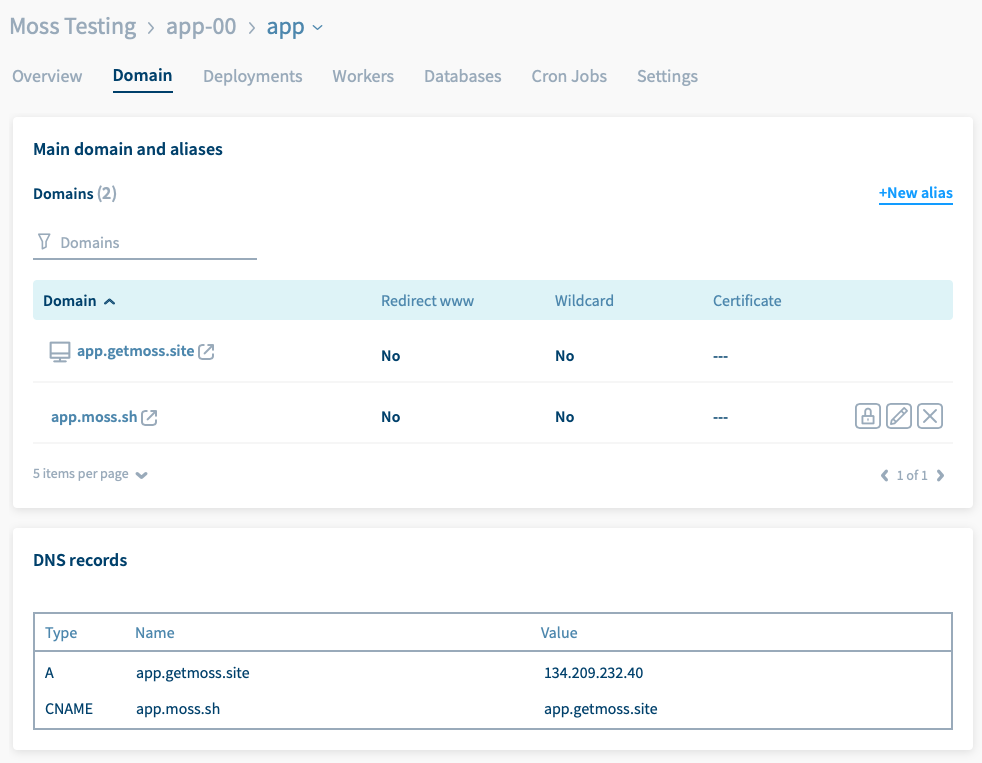The graphic illustrates a white-backed web interface labeled "Moss Testing" at the top in gray font, accompanied by a right-pointing arrow. It includes "app-00," followed by another gray arrow, leading to "app" displayed in blue with a corresponding drop-down arrow beside it. At the top section, various tabs are visible: "Overview" in gray, and "Domain" highlighted in blue, underlined with a blue line. Other tabs such as "Deployments," "Workers," "Databases," "Cron Jobs," and "Settings" are also listed in gray.

Below, the interface shows "Main Domain and Aliases" and "Domains (2)" highlighted in blue. There is a "New Alias" button with a plus sign, underlined and colored light blue to the right. The "Domain" header appears on a blue band or header, displaying options such as "Redirect," "www," "Wildcard," and "Certificate."

At the bottom, the section for "DNS Records" is present, detailing different record types including a type "A" record with its respective name and value, and a type "CNAME" record with its own name and value. This structure provides a comprehensive view of the domain management dashboard.